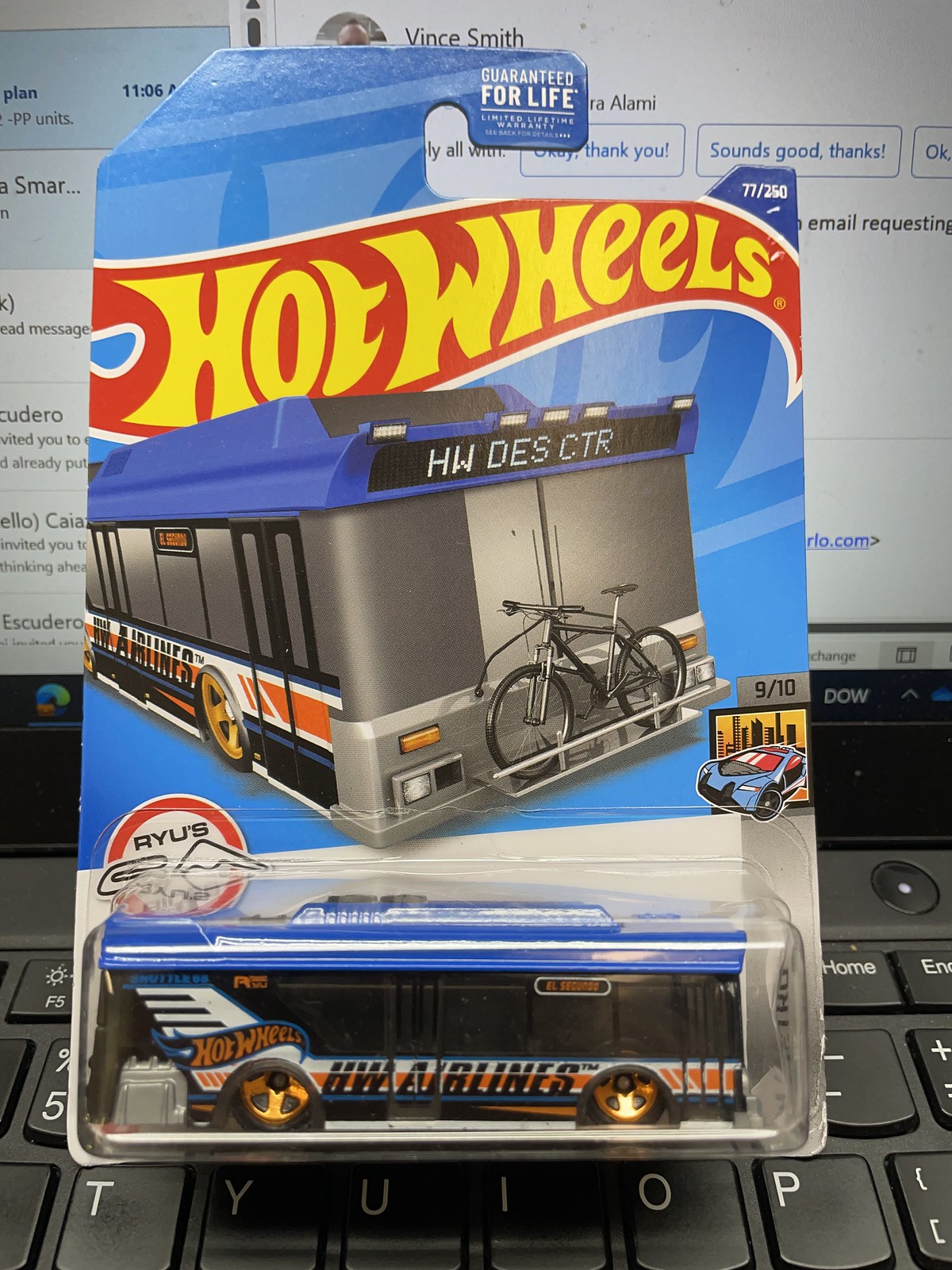The image showcases a detailed Hot Wheels bus toy encased in a mixed plastic and paper packaging designed for display, featuring a hook area labeled "Guaranteed for Life" at the top, with a "Limited Lifetime Warranty" noted to the right. The top right edge of the packaging also displays "77/250." Prominently, the Hot Wheels banner is centered at the top with "hwdsctr" printed below it. The bus toy itself, branded as "Hot Wheel Airlines," is depicted twice: once in the packaging illustration showing a stylized bus coming towards the viewer with a little bike on the front, and again as the physical toy inside the casing. This toy bus, adorned with red and white striped wheels, features non-transparent yellow windows and sports a blue and black color scheme. Additionally, there's a small airplane wing detail on the back left side of the bus. In the background, a black laptop is visible, with an open email from a sender named Vince Smith, adding a personal touch to the scene.